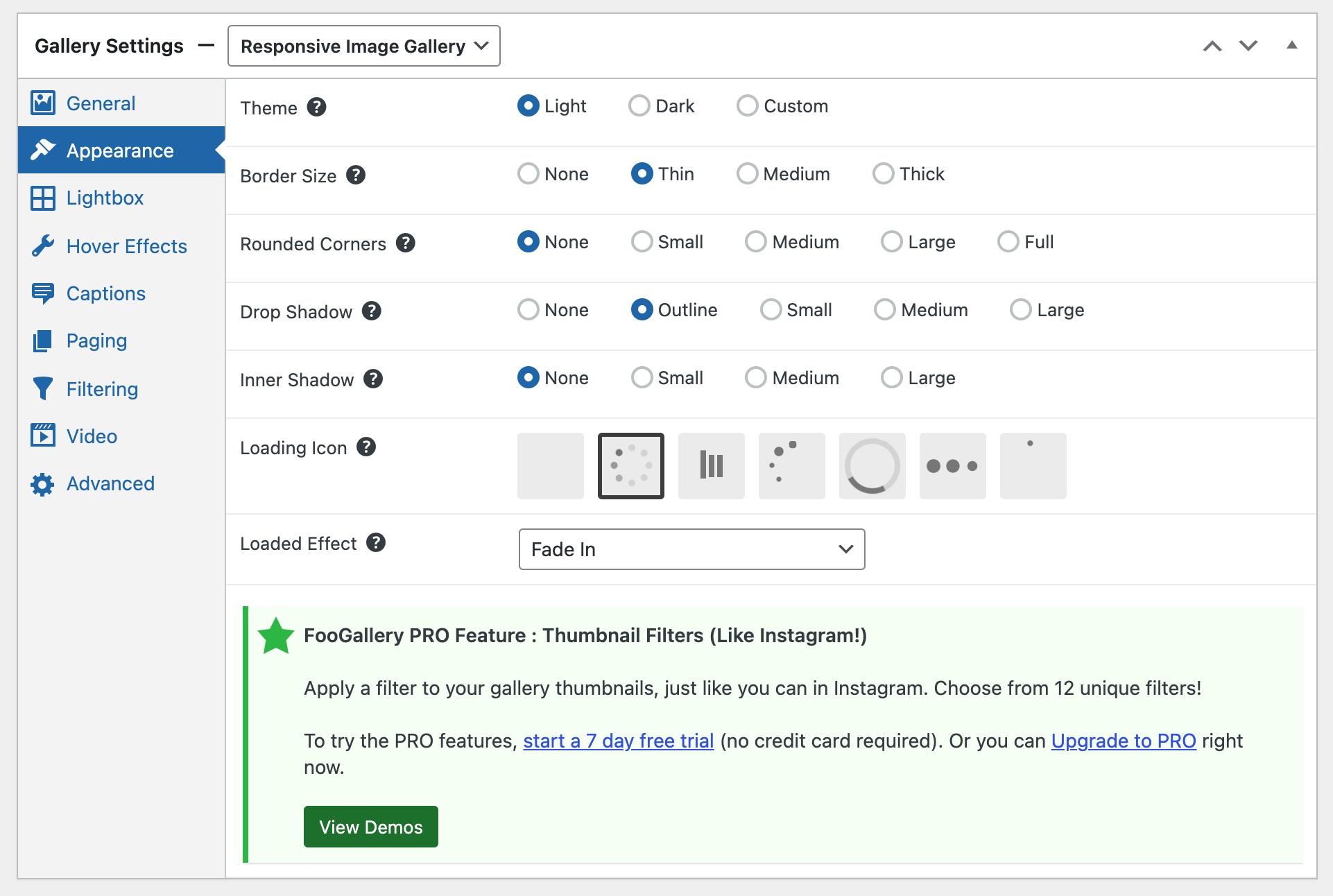Screenshot of the webpage extends from the top to the bottom, detailing various settings and options for an image gallery. 

At the top, from left to right, the header reads "Gallery Settings." Adjacent to it, on the right, it displays "Response Image Gallery" followed by a responsive image gallery options menu. Next to this, there's a dropdown menu accompanied by up and down arrows, with an additional up arrow situated at the far right.

The left sidebar lists categories in a vertical column, including:
- General 
- Appearance 
- Lightbox 
- Hover Effects 
- Captions 
- Paging 
- Filtering 
- Video 
- Advanced (marked with a sprocket icon).

To the right of the sidebar, the main settings interface is divided into sections. It begins with the "Appearance Theme" settings across the top:
- The "Theme" selection shows "Light" checked (active), while "Dark" and "Custom" remain unchecked.

The next section down covers "Border Size:"
- "None" is not checked.
- "Thin" is checked.
- "Medium" and "Thick" are not checked.

Further down, "Rounded Corners" options display:
- "None" is checked.
- "Small," "Medium," "Large," and "Full" are not checked.

For "Drop Shadow:"
- "None" is unchecked.
- "Outline" is checked.
- "Small," "Medium," and "Large" are unchecked.

Moving to "Inner Shadow:"
- "None" is checked.
- "Small," "Medium," and "Large" are unchecked.

In the "Loading Icon" section, several selection boxes are visible:
- The first box is unchecked.
- The second box, represented with a circle icon, is checked.

Finally, "Load Effect" settings show a dropdown menu:
- "Fade In" is selected within the dropdown menu.

This detailed visual arrangement of options provides comprehensive configuration for optimizing the appearance and functionality of the image gallery.